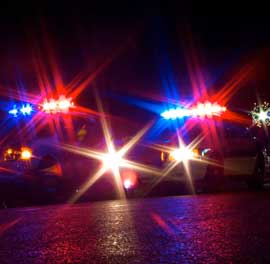In this nighttime photograph, a group of police cars appears to be moving toward the photographer on a shiny, possibly rain-slicked roadway. The scene is bathed in an array of flashing red, blue, and green emergency lights, creating a blurred and intense visual effect. While it’s challenging to determine the exact number, estimates suggest there are up to eight or nine police vehicles involved. The darkness of the sky contrasts starkly with the bright headlights and strobing first response lights, adding to the urgency of what seems like a rescue or emergency situation. The presence of additional light sources, possibly streetlights, enhances the pavement reflections, further underscoring the dramatic and chaotic nature of the scene.